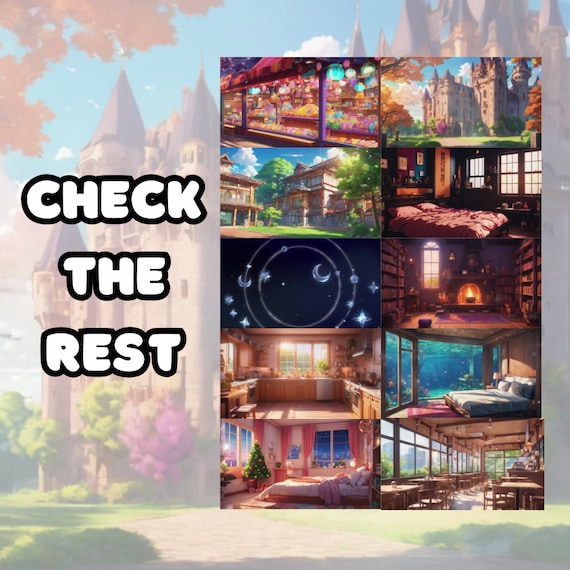This is an advertisement postcard for Disneyland accommodations, prominently displaying the message "Check the rest" in white letters with a black outline on the left-hand side, partially covering a faint image of the iconic castle in the distance. The card features eight small, vividly detailed photos of different themed bedrooms and environments, resembling a blend of bungalows with unique celestial decors and traditional rooms. One bedroom has a cozy fireplace flanked by bookshelves, with a fire crackling warmly in the hearth. Another room showcases a serene pink-themed decor, complete with pink curtains, white bed covers accented by a pink blanket, and a charming green Christmas tree adorned with round ornaments. Among these images is a captivating celestial-themed room, depicting rings around moons and scattered stars against a black sky. Additionally, there's an image suggesting a delightful candy shop or kitchen, potentially offering baked goods, enhancing the cozy and inviting atmosphere of this proposed vacation destination.